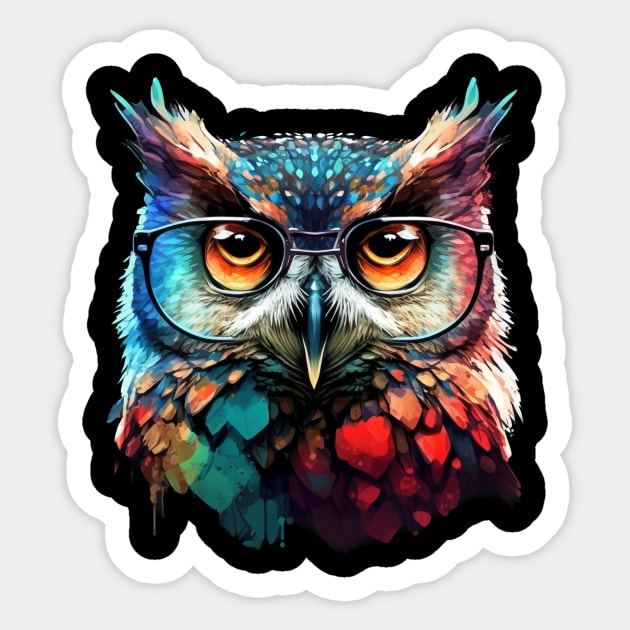This is a photograph of a vibrant and whimsical sticker featuring a detailed drawing of an owl with fantastical feathers. The owl, wearing reading glasses perched on its sharp beak, presents a colorful and captivating appearance. The top of its head is adorned with blue feathers, and purple feathers extend above its glasses. The owl's eyes are a striking combination of orange and yellow, giving it a stern, perhaps annoyed look. Its feathers boast a vivid mix of turquoise, green, orange, red, and varied shades of blue. The left side of its face is highlighted by blue feathers with hints of peach-red, while the right side exhibits red, orange, and white feathers. The entire image is bordered by a black outline followed by a white one that contours the owl's head, set against a light gray background. This fun and decorative sticker, perfect for adorning a notebook or other items, stands out in the center of the photo.